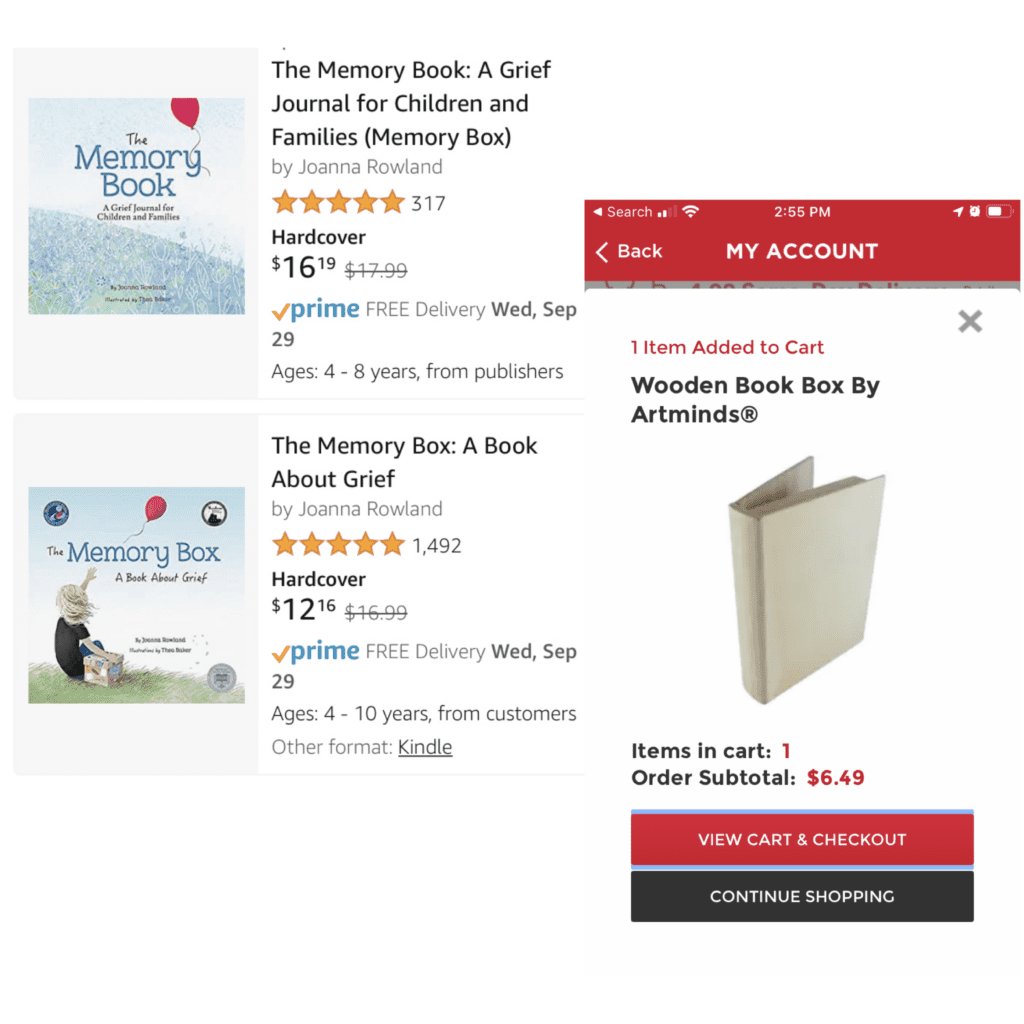The image showcases two listings from an Amazon page featuring books about grief for children and families. 

On the left, the first listing is for "The Memory Book: A Grief Journal for Children and Families" by Joanna Rowland. The cover image, set against a gray background, depicts a sky and possibly a hillside with a red balloon floating away. The book's title is written in blue, with additional details in black text beneath it. To the right of the image, the listing displays the book's full title, author, and details: it has received a five-star rating from 317 reviews. The hardcover price is listed at $16.19, with the original price of $17.99 crossed out. It also includes the Prime logo with a note for free delivery by Wednesday, September 29th, and is suitable for ages four to eight years.

Below this, the second listing on the left features "The Memory Box: A Book About Grief," also by Joanna Rowland. The cover illustration depicts a young girl sitting on a grassy hill, releasing a red balloon, with two stamp logos in the upper corners. The listing indicates the book has a five-star rating from 1,492 reviews. The hardcover version is priced at $12.16, reduced from the original price of $16.99, and also includes the Prime logo with free delivery promised by Wednesday, September 29th. This book is recommended for children aged four to ten years and is available in other formats, including Kindle.

To the right of the listings, there is an overlay showing a screenshot from a cell phone. The red bar at the top includes a search option, signal indicators, Wi-Fi logo, the current time (2:55 PM), location icon, alarm clock icon, and battery life status. Below this, a white box indicates that one item has been added to the cart: a "Wooden Book Box" by Art Minds, priced at $6.49. The cart summary shows one item with a subtotal of $6.49. There’s a red button labeled "View Cart and Checkout" and a black button labeled "Continue Shopping."